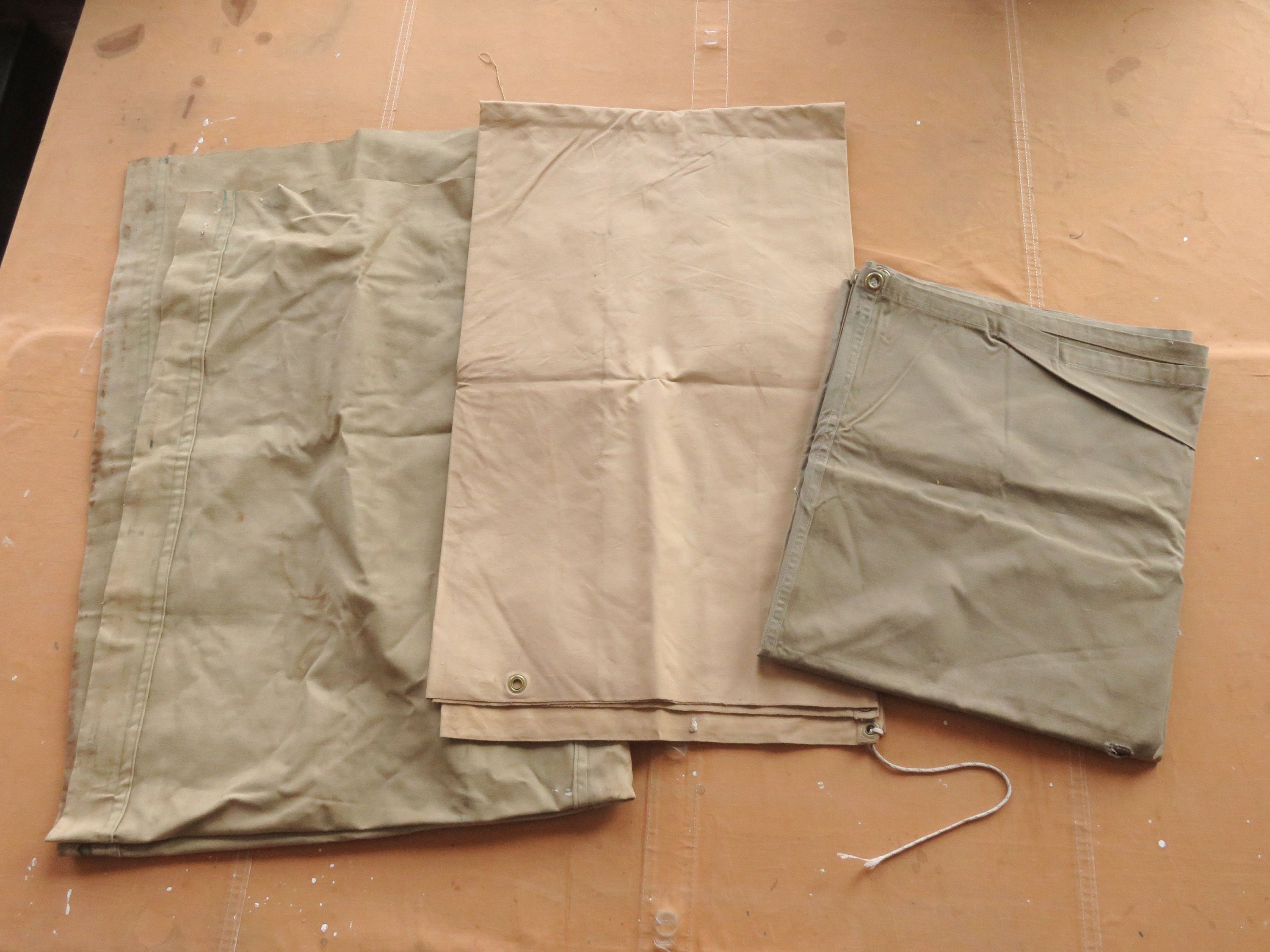The photograph displays an arrangement of canvas-like fabrics on an orange, stitched table covering. On the left is a large, wrinkled, light green fabric folded into a sizable rectangle. Adjacent to it in the center, a smaller peach-pinkish khaki fabric is folded into another rectangle, featuring multiple grommets along its bottom edge and a piece of string that's partially torn. On the right is a darker, army green fabric, folded into a near-square, significantly smaller than its counterparts, with a single visible grommet. Each of these materials bears characteristics of being worn and creased, suggesting they might be drawstring bags or parts of sails. They all rest atop a substantial, brownish canvas-like tarp.